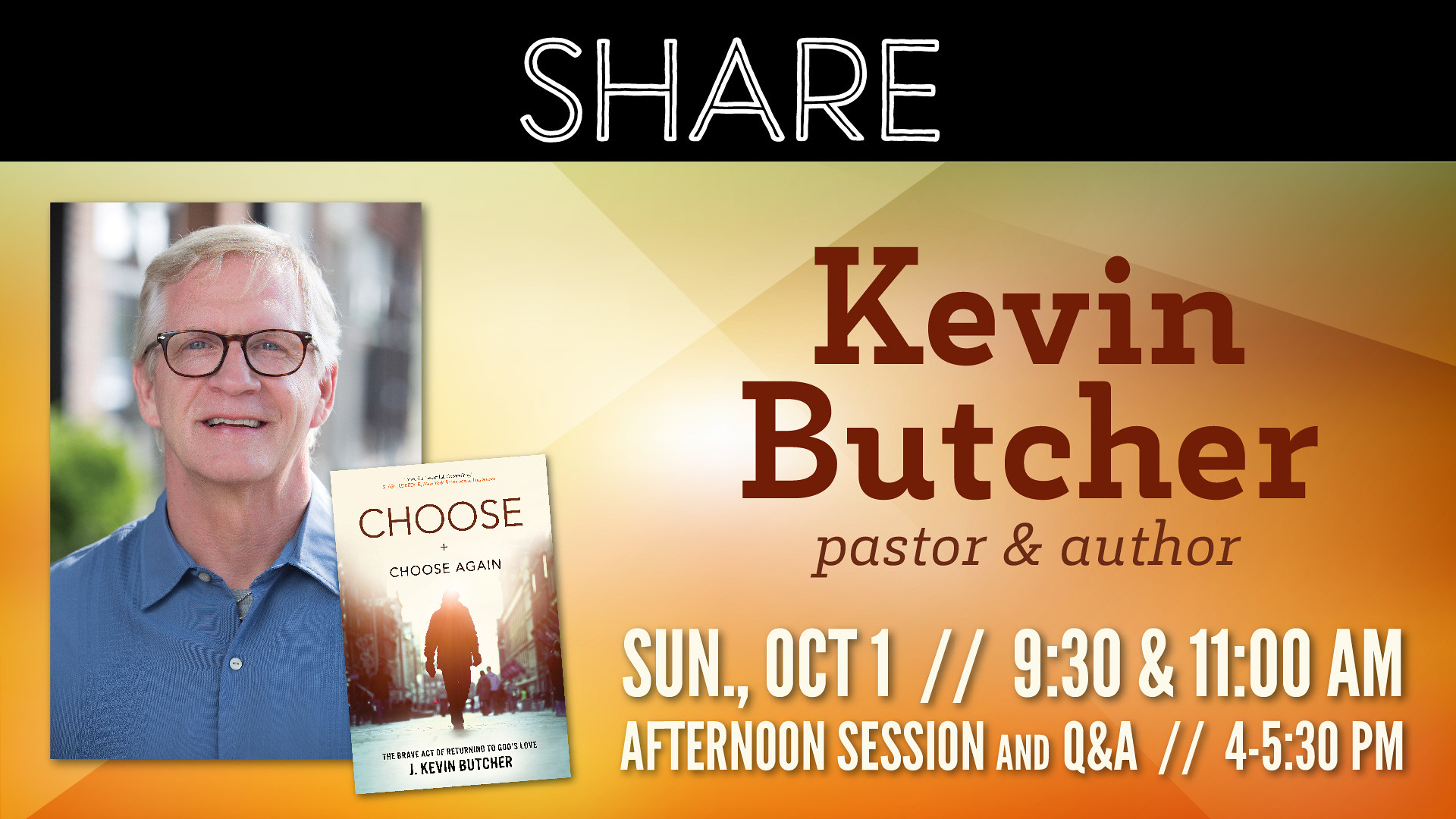The image appears to be an advertisement for a book promotion event featuring Pastor and Author Kevin Butcher. The top of the image features the word "Share" in white font against a black background. Below this, the background transitions to an orange and yellow geometric pattern. Prominently displayed is a portrait of Kevin Butcher, a man with white hair, wearing dark glasses and a blue collared shirt. To the right of his photo, "Kevin Butcher, Pastor and Author" is written in large brown letters. Below this, event details are listed: "Sunday, October 1st, 9:30 and 11 a.m., Afternoon Session and Q&A, 4 to 5:30 p.m." Overlapping the corner of his portrait is an angled image of his book cover titled "Choose and Choose Again," featuring a silhouette of a man walking along a street. This detailed ad promotes his upcoming presentation and book signing event.